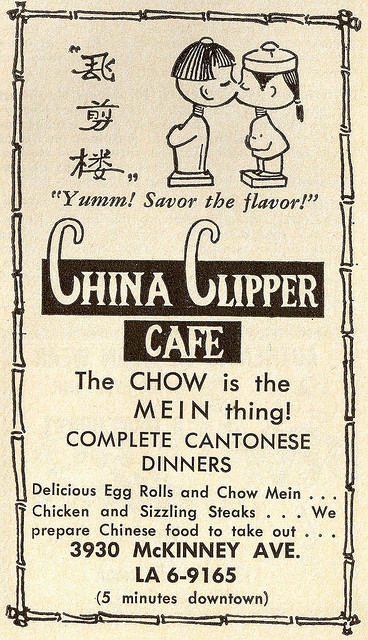This advertisement for the China Clipper Cafe is printed on pale pink paper, accentuated by a black ink border designed to resemble sticks of bamboo. At the top, a series of Chinese characters are displayed vertically. Below this, a charming illustration of a young man and woman, depicted in a simple cartoon style, captures them leaning in to share a kiss. Accompanying this image is the exclamation "Yum! Savor the Flavor!" in playful lettering.

A prominent black banner with light pink letters proudly announces the cafe’s name: China Clipper Cafe. Just beneath, the slogan "The chow is the main thing" cleverly plays on words, using "main" spelled as "M-E-I-N" to reference the staple noodle dish.

Further details in smaller black text boast about the cafe’s complete Cantonese dinners, highlighting popular dishes such as "delicious egg rolls and chow mein, chicken, and sizzling steaks." The message assures potential customers that they also prepare Chinese food to take out.

Finally, the advertisement provides the cafe's address in bolder black letters, with an added note in parentheses indicating it is only "five minutes downtown."